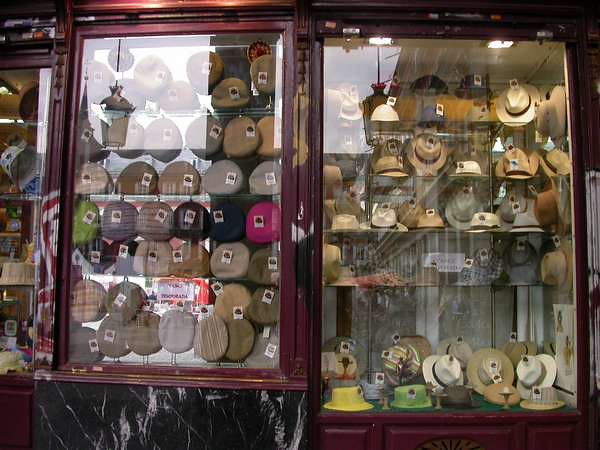The image showcases a charming, old-school storefront with a focus on its window display, framed by a mahogany, red-brown wood exterior on one side and a black and white, marble-hued facade on the other. Prominently, there are two detailed display cases filled with a variety of hats. On the left, the display case, partially cut off, features Scallywag-type hats, reminiscent of the 1940s mailman style, each accompanied by a price tag. The base of this case exhibits a striking black marble pattern. In the center, another display case stands with an array of berets in different colors, from neutral tans and soft greens to vibrant lime greens and pinks, resting on a black marble base. The right section of the image reveals a large display case brimming with Fedora-style hats and possibly top hats, many adorned with decorative straps just above the brim. The hats vary in color, predominantly white and cream, with standout pieces in yellow and green. This display case, extending from the middle to the right side of the image, is set on a maroon base and showcases each hat with individual tags, all under gleaming, glary glass covers that reflect a light source. This meticulously arranged storefront seemingly caters to an array of traditional men's headwear.